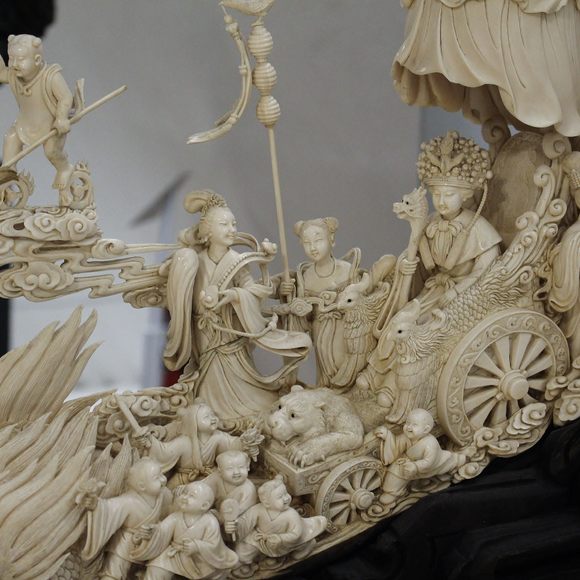The image depicts an intricate, ivory-colored Chinese carving that exudes opulence and attention to detail. Central to the carving is a grandiose chariot, ornately decorated with dragon motifs and intricate designs on its wheels. Riding in the chariot is an empress, distinguished by her lavish floor-length dress, a scepter adorned with a dragon's head, and a regal crown. Accompanying her are two women who appear to be servants, highlighting the hierarchical structure. Surrounding the chariot are various animals and cherubic figures, adding layers of complexity and luxury to the scene. The empress looks happy and content, in contrast to the more neutral expressions of those around her. The overall composition of the carving showcases the excess and opulence of royal life, with numerous babies carved into the scene, symbolizing fertility or prosperity.